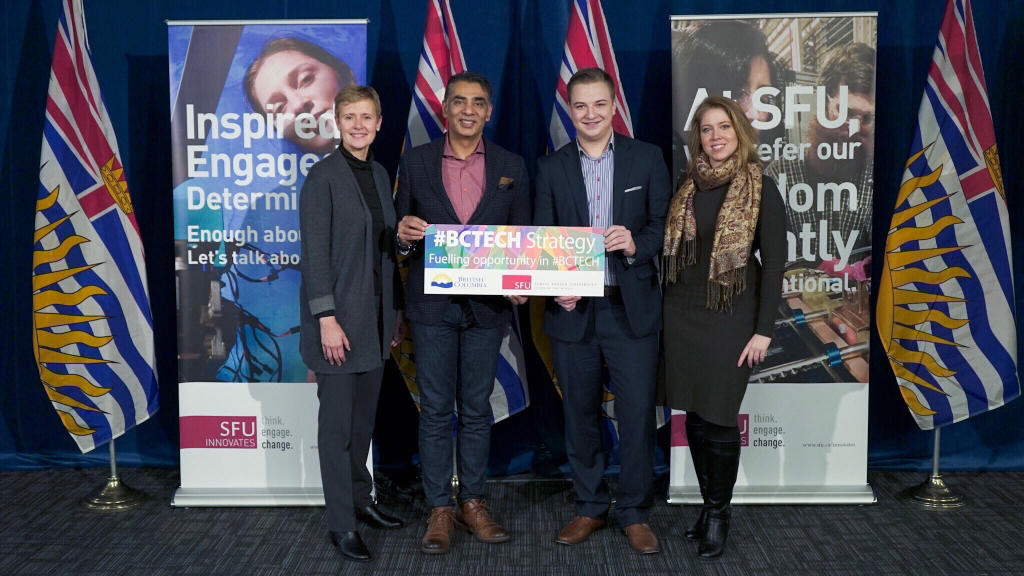Four formally dressed individuals stand in a line in front of a backdrop featuring posters, flags, and logos. The two women are positioned on the outer edges, with the two men in the center, both wearing suits and holding a sign that says "#BCTechStrategy fueling opportunity in #BCTech." The sign also displays logos for British Columbia and SFU (Simon Fraser University).

The man to the left in the center is wearing a pinstripe blue shirt under his dark suit and appears to be a white gentleman smiling toward the camera. Next to him stands a younger South Asian man in a maroon shirt, also smiling. To their left is a woman with short dirty blonde hair, dressed in a gray pantsuit, exuding a professional demeanor. On the far right is another woman with shoulder-length hair, wearing a black turtleneck under a gray cardigan paired with gray slacks and short boots.

Behind the group, various flags with blue and white stripes and sun symbols can be seen on flagpoles. Two large freestanding posters flank the quartet: the left one features the words "Inspired, Engaged, Determined" and a mention of "SFU Innovates: Think, Engage, Change," while the right poster prominently displays "SFU" in white text. These visual elements collectively highlight the theme of innovation and technology, reinforcing the significance of the BC Tech Strategy event.